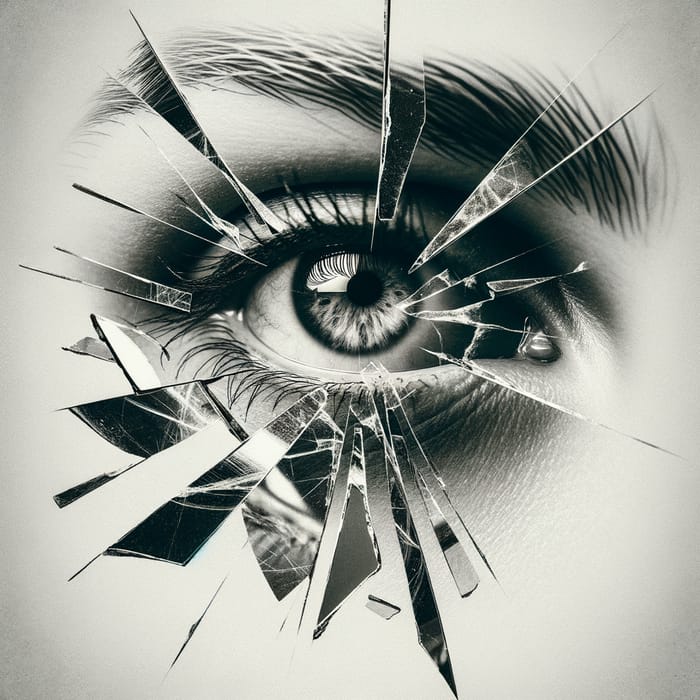This is a highly detailed, black and white image of a close-up of a person's right eye. The artwork appears to be meticulously done, likely with pencil, capturing an impressive level of realism. The eye is heavily accentuated with makeup, including mascara, eyeliner, and eyeshadow, suggesting it could be a woman's eye due to the soft features and cosmetic detailing. The dark eyebrow slants down to the right, further indicating it is the right eye. The eye itself is glistening, revealing fine details such as the pupil and the intricate reflections on the eyeball. Surrounding the eye are fragments of shattering glass, adding a surreal element to the composition. These shards reflect minute details from the eye and its surroundings, enhancing the overall impression of meticulous craftsmanship. The realistic portrayal extends to individual strands of hair in the eyebrow and eyelashes, emphasizing the incredible detail and artistry of the image.